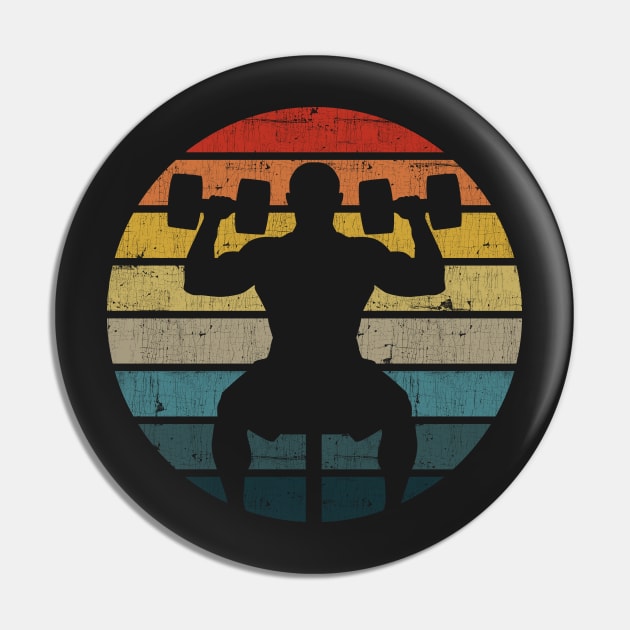The image portrays a striking piece of digital art resembling a logo or decorative wall sign. The background is a subtle grey, but the focal point is a black, circular frame that holds the central artwork. Inside this circle, a powerful silhouette of a muscular, bald man sitting on a weightlifting bench is seen from behind. His bare upper body and biceps are well-defined as he lifts two dumbbells to shoulder level, creating an 'L' shape with his arms. The silhouette is set against a vibrant, horizontal gradient, composed of eight colored stripes that transition smoothly from red at the top through orange, yellow, greenish-gray, blue, blue-green, and finally to dark blue at the bottom. Each color strip takes up a small section of the image, creating the illusion of a rainbow spectrum as the black silhouette stands prominently in the foreground. The overall effect is both striking and colorful, making it look like a badge or emblem meant for decor.